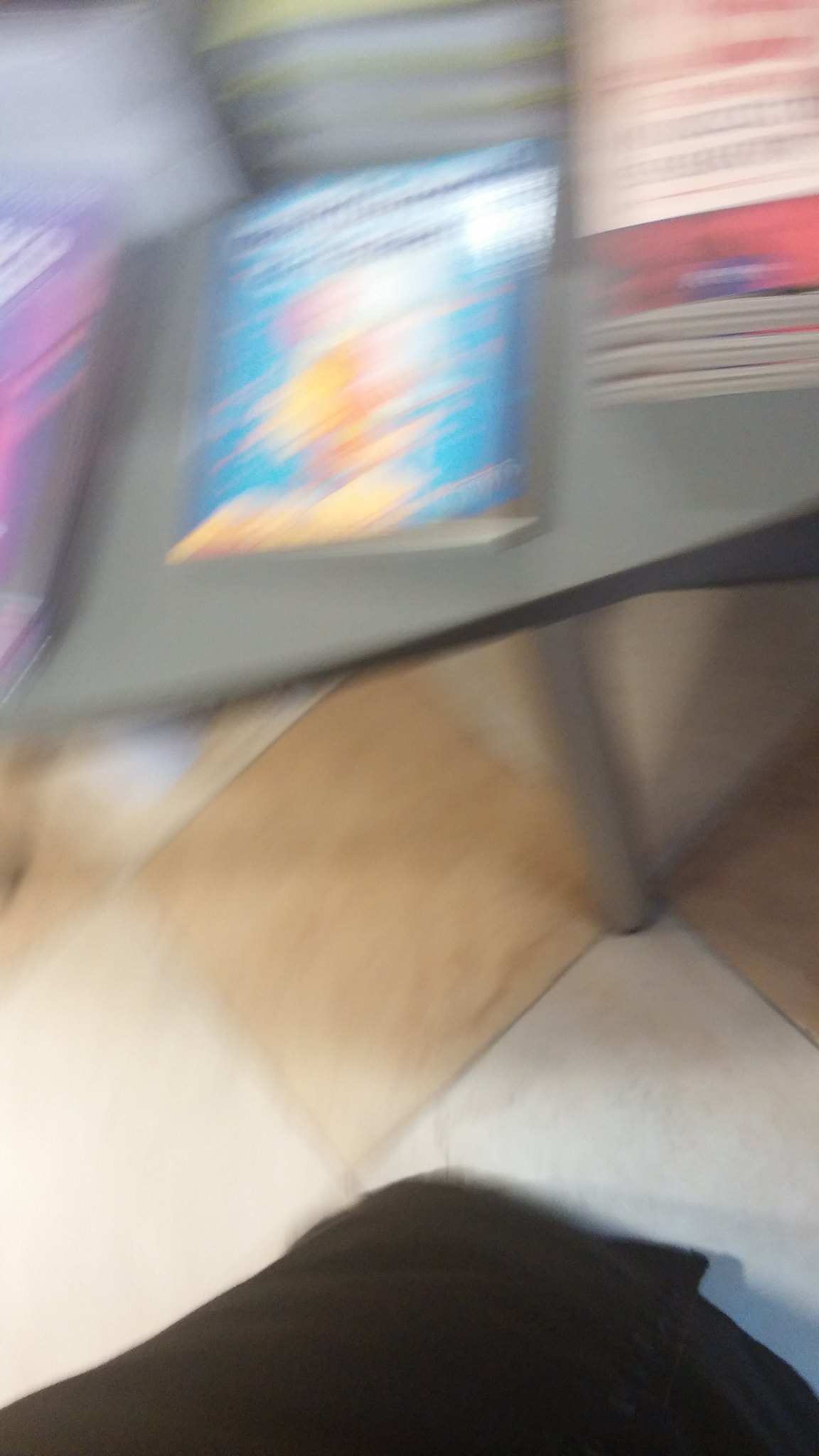The photograph is extremely blurry, as if the person taking it was spinning in a circle. It is roughly two and a half times taller than it is wide. The bottom portion reveals a checkered tile floor with equilateral, diamond-shaped tiles alternating between medium brown and light brown (or a pale cream and a dark cream beige in a checkerboard pattern, depending on interpretation). In the lower section of the image, there appears to be a leg or body part draped in a long black skirt or pants. The top half of the image features a grey table with round silver legs, running from left to right across the image. On the left end of the table is a teal item—possibly a DVD case or a book—with yellow and orange details near its center. Additionally, there are stacks of books or pamphlets on the table, including red, blue, pink, purple, and possibly green or white ones. However, due to the blur, the exact details of these items are indistinguishable.